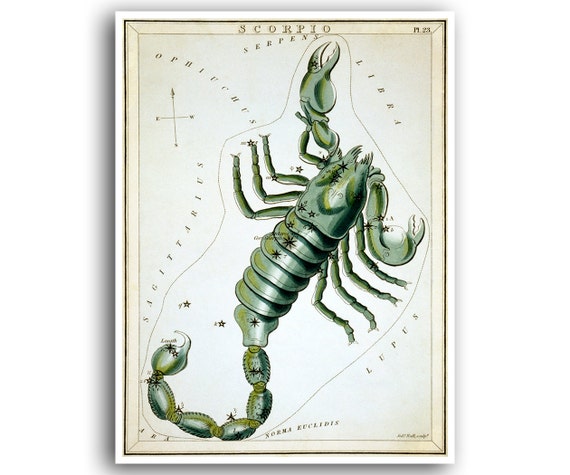In this photograph, we see a framed astrological artwork featuring the sign of Scorpio. The frame is white, and the center of the image has an aged paper look with a yellowish-ivory tone, set against a pale bluish background. Dominating the center is a detailed drawing of a large green scorpion in a diagonal position, with its segmented body, claws, legs, and a curly tail that wraps around the bottom of the image. The top of the artwork prominently features the word "Scorpio," with other astrological names such as Sagittarius, Libra, Serpens, Ophiuchus, Era, Norma, Euclides, and Lupus arranged around the scorpion. Additionally, a north, south, east, west symbol is present, and small stars are interspersed around the drawing, adding to the celestial theme.